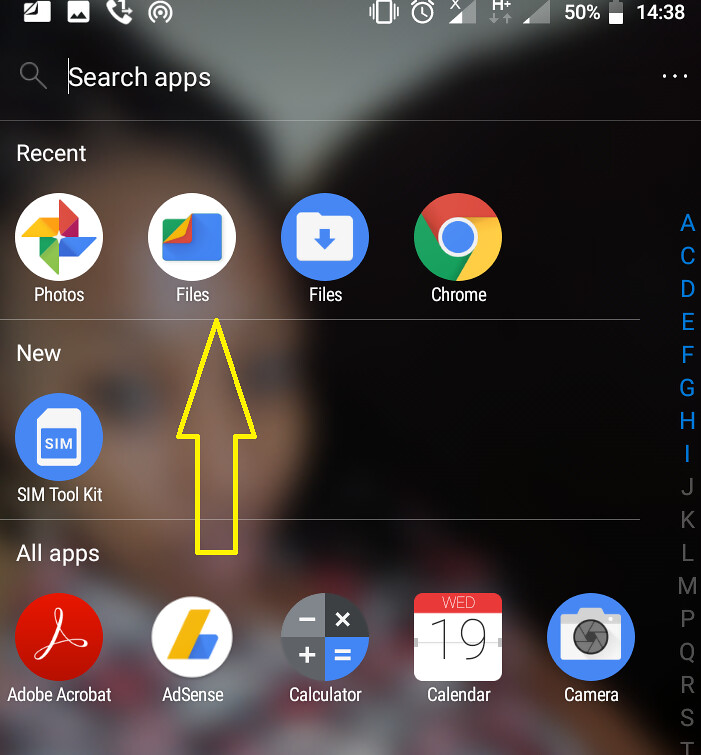The image displays a smartphone application screen with detailed UI elements. At the top of the screen, small white icons indicate various system statuses. The battery icon shows a 50% charge level, and the time is displayed as 14:38. Below the status bar, there is a search area highlighted by a magnifying glass icon and the text "Search apps."

Further down, a horizontal section labeled "Recent" shows a selection of recently used applications, including Photos, Files, Files, and Chrome. Beneath this, another horizontal section titled "New" features a blue circle with text "SIM" and an application named "SIM Toolkit" underneath it.

At the bottom, the screen has a section labeled "All Apps," displaying icons for Adobe Acrobat, AdSense, Calculator, Calendar, and Camera. Separating these horizontal sections, there is a yellow upward-pointing arrow. This arrow starts in the bottom panel and extends to the top panel, slightly left of the center of the screen.